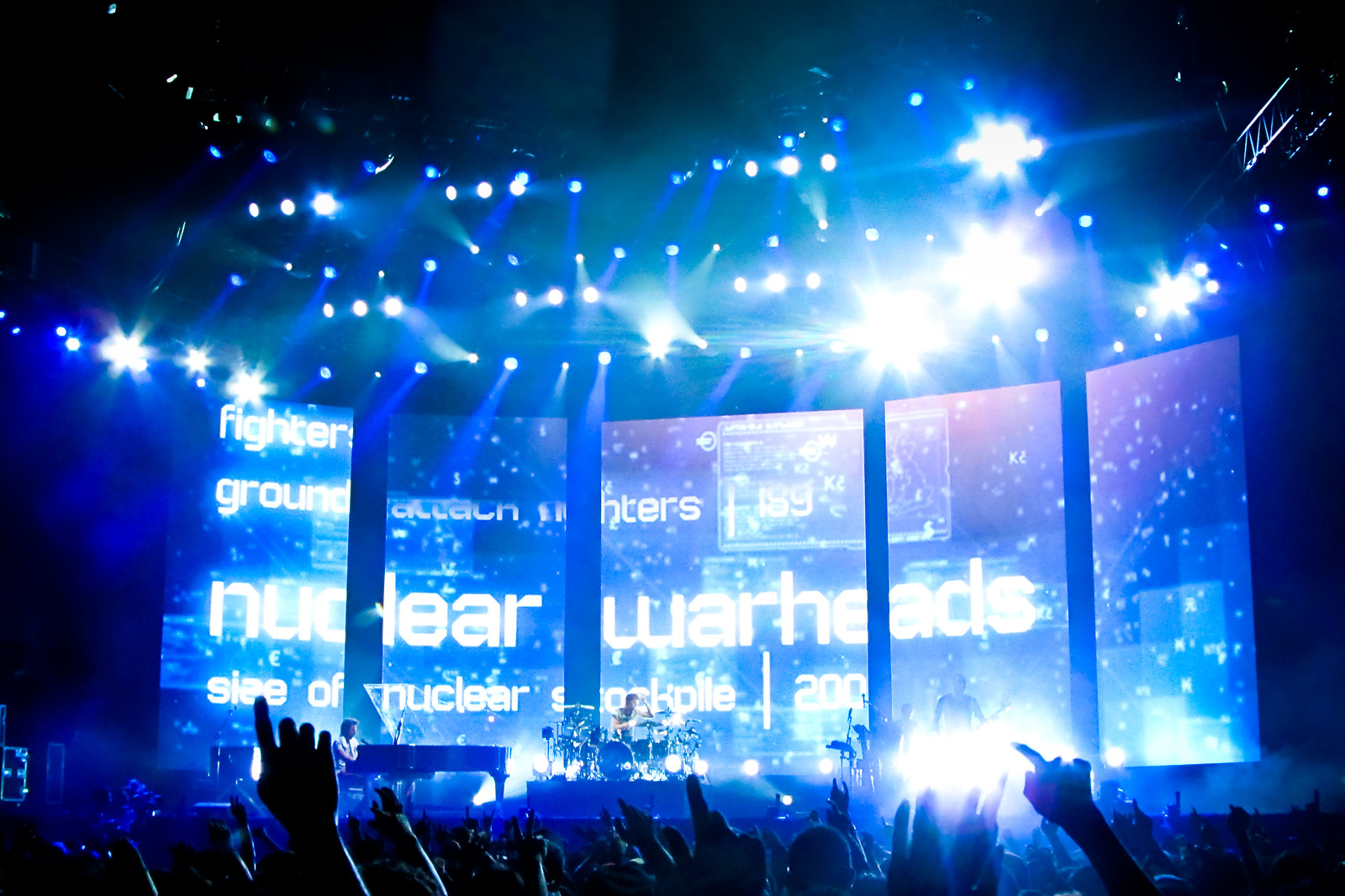This photograph captures the exhilarating atmosphere of a large indoor concert from the vantage point of the audience. The venue is massive, with four prominent pillars framing the scene and an overall majestic and grand feel. The expansive stage is bathed in a sea of brilliant blue and white lights that illuminate the entire space, giving it a magical aura. 

At the center of the action, a band is performing energetically, with a grand piano stationed on the left side of the stage being played by a man in a white shirt. Towards the middle, a drummer is commanding a large drum set perched on a riser, while to the right, a guitarist can be seen, though the bright lights make it a bit challenging to discern details.

The backdrop of the stage features a series of vertical screens that merge into one enormous horizontal display. The screens are awash in blue hues, with digital effects and falling confetti, and prominently feature white text that reads "fighter ground nuclear warheads." Additional words like "stockpile" are partially visible, adding to the dramatic visual setting.

In the foreground, the enthusiastic crowd is fully engaged, with many audience members raising their hands, creating a lively sea of shadows and silhouettes against the vibrant lights. At the top of the image, stage lighting rigs with circular lights cast a bluish glow over the entire concert, further enhancing the electric atmosphere. Attendees are clearly enjoying the show in this beautiful and captivating venue.